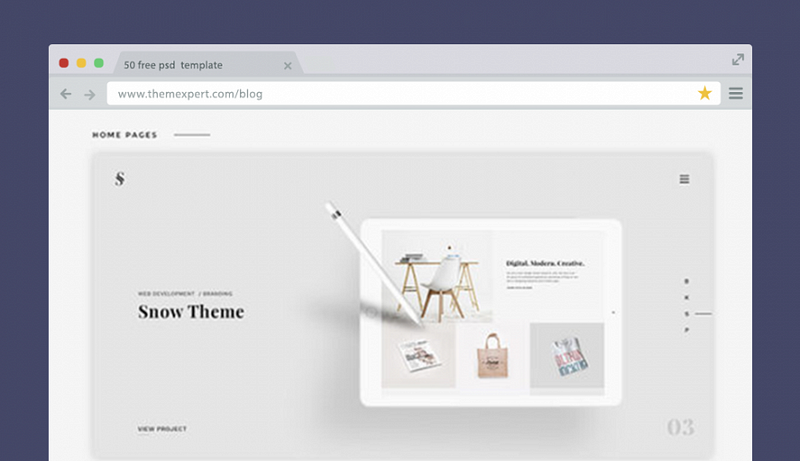This image captures a detailed view of a web browser interface featuring a variety of elements. In the top left corner, there are three circular buttons colored green, yellow, and red. Although the specific browser is not identified, the visible tab displays the text "50 free PSD templates." Directly beneath the tab, there are back and forward navigation arrows, as well as a web address bar showing the URL "www.themexpert.com/blog." Below the address bar, the webpage content begins with the heading "Homepages," accompanied by a horizontal line extending to the right. Dominating the main section of the webpage is a large gray box, located centrally. In the top left corner of this gray box is an 'S' symbol. Towards the center-left of the gray area, the words "Snow Theme" are displayed prominently. Adjacent to this, on the right side, is a white box featuring an illustration of a pen writing on a tablet.